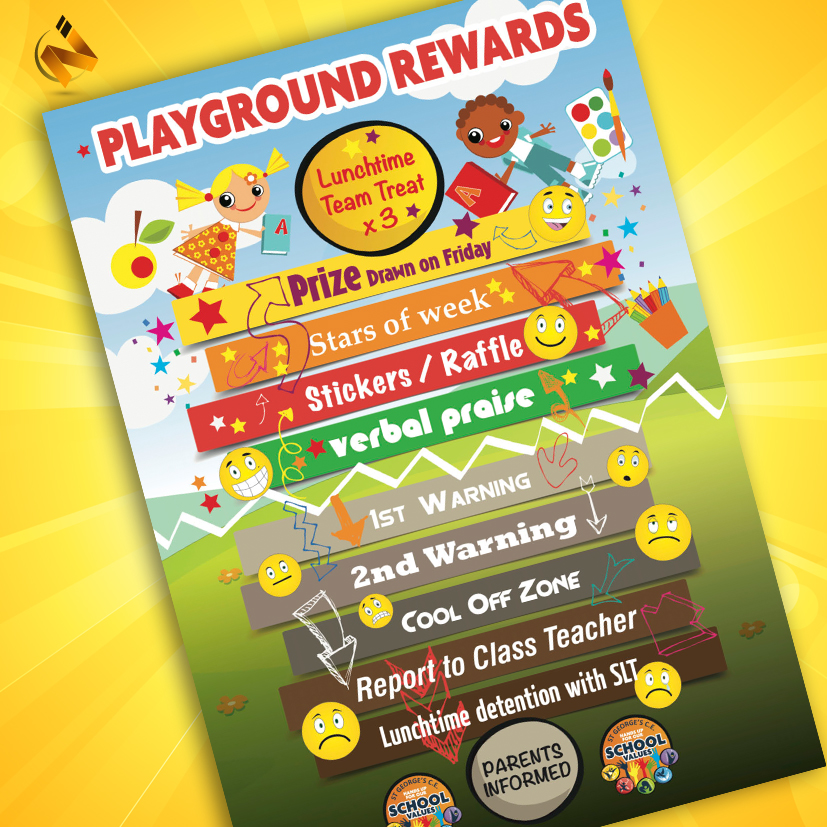The image illustrates a colorful and detailed sign titled "Playground Rewards," clearly designed for children and their parents. The background is a bright yellow, creating an engaging and visually appealing display. At the top of the sign, the heading is prominently displayed in colorful and cartoony text. Surrounding the title are cheerful cartoons of a girl on the top left and a boy on the top right, each holding books, which adds a playful touch to the design.

The sign outlines a reward and disciplinary system for playground behavior, detailed as follows:
- **Lunchtime Team Treat x3**: Rewards for positive behavior during lunchtime, indicated likely by three opportunities.
- **Prize Drawn on Friday**: A chance for well-behaved children to win prizes.
- **Stars of the Week**: Recognition for exemplary behavior.
- **Stickers/Raffle**: Additional incentives for good conduct.
- **Verbal Praise**: Immediate acknowledgment for positive actions.

For misbehavior, the chart shows a descending order of consequences:
- **1st Warning**: Initial alert to correct behavior.
- **2nd Warning**: Follow-up warning if behavior does not improve.
- **Cool-Off Zone**: Temporary removal from activities to calm down.
- **Report to Class Teacher**: Escalation if previous steps are ineffective.
- **Lunchtime Detention with SLT**: More serious consequence involving the Senior Leadership Team and detainment during lunch.
- **Parents Informed**: Notification to parents regarding their child’s behavior.

To visually support the text, the sign includes various emojis ranging from smiley faces for positive actions to unhappy and scared faces for negative behaviors, making it easy for children to understand the implications of their actions. The layout is clear and organized, with the rules and rewards easily readable.